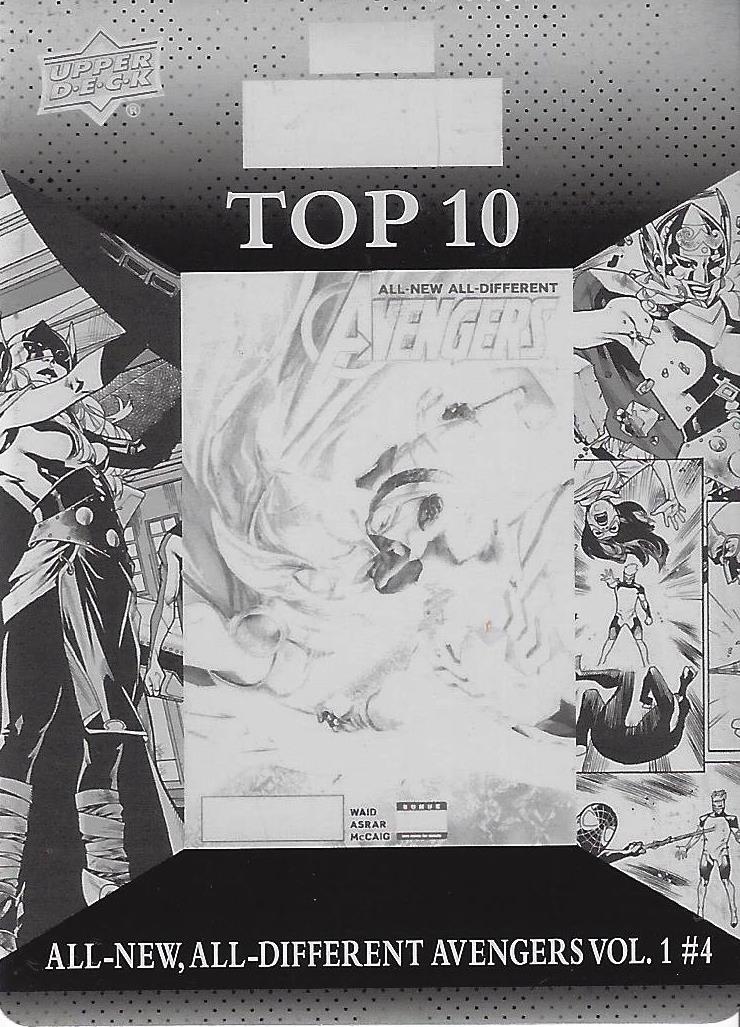This is a black-and-white image featuring what appears to be a comic book cover or a card with comic book elements. At the top of the picture, there is a gray area dotted with black spots indicating "Top Ten," and to the left, the "Upper Deck" logo is visible. The central part of the image is dominated by the cover of "All New, All Different Avengers," which is slightly faded but still readable. Surrounding the main cover are various black-and-white cutouts depicting animated scenes and characters, including recognizable figures like Spider-Man and possibly members of the X-Men. On the left side, there is a depiction of a female character, and on the right, additional scenes illustrating characters, including one of a character falling. At the bottom of the image is a black hexagon shape with the text "All New, All Different Avengers Volume One, Number Four" written in white letters. The overall composition suggests a visual representation of multiple Marvel characters and scenes, brought together in a monochromatic, collage-like fashion.